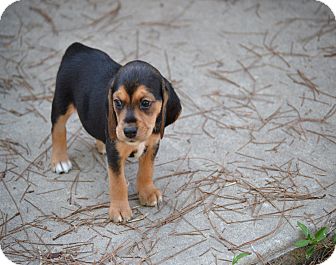This image features a small puppy with predominantly black fur that transitions to tan on its legs and face, and highlights of white on its chest and toes. The black fur on its head forms a distinct triangle that leads down to its black nose, and it has black floppy ears. The puppy, which appears a bit sad, is looking off to the left while standing on a piece of gray cement. The concrete surface is scattered with dried pine needles, and in the bottom right corner, a patch of greenery with a weed peeks through. The scene captures the puppy in a contemplative pose amidst the subdued tones of its surroundings.